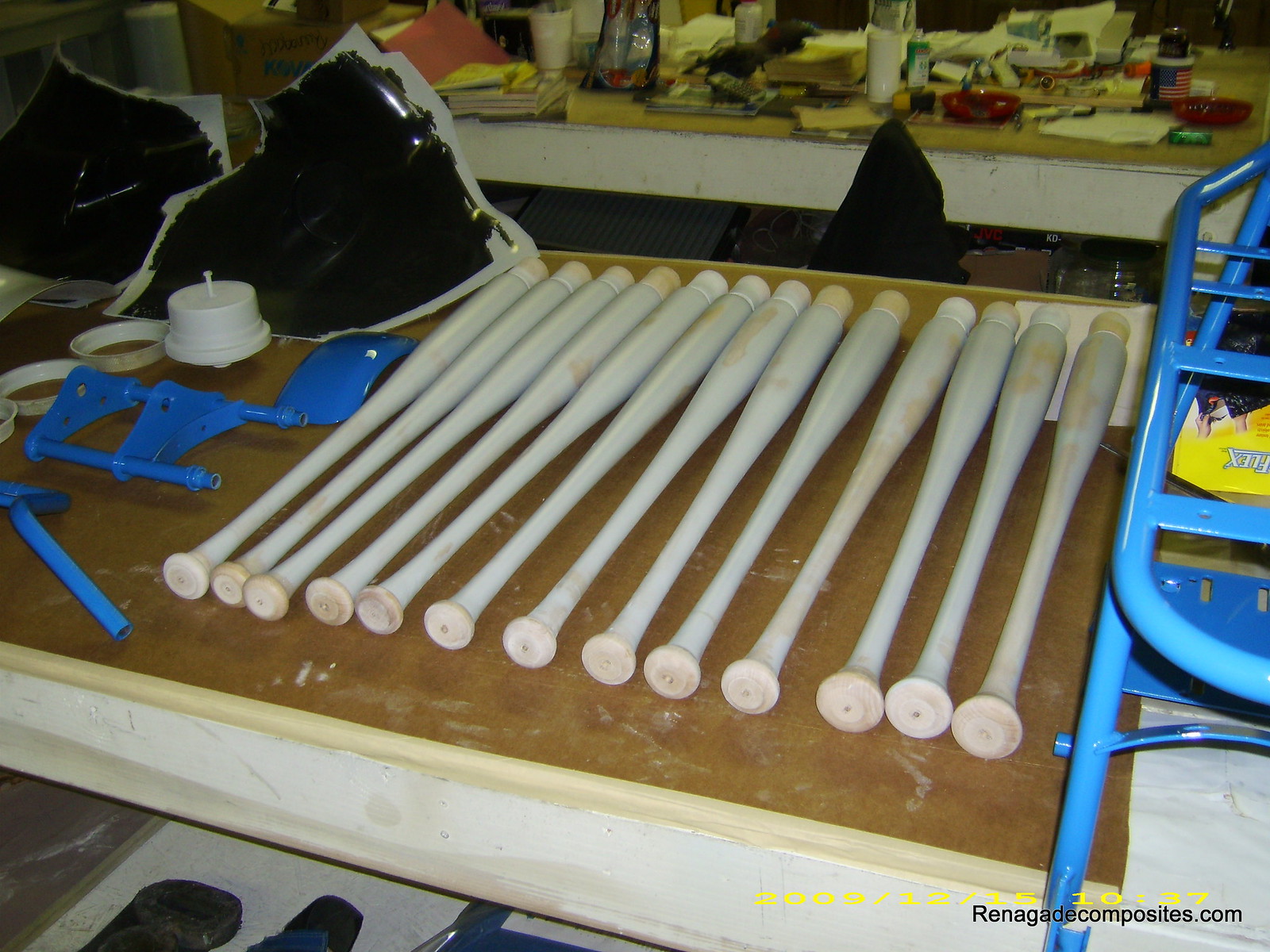The image depicts a bustling factory workspace dedicated to assembling various baseball-related items. Central to the scene is a rough, tan wooden table edged with a white border, where approximately 15 white baseball bats are meticulously lined up side by side. Splashes of white paint can be seen on both the bats and the table surface, suggesting recent craftsmanship. The table is cluttered with various tools and components, including a black and white guard-like object, numerous metal and plastic parts, and a triangular structure with a pipe, all glossy blue in color. In the background, another tan table, also with a white border, is loaded with an assortment of styrofoam cups, plates, papers in pink, yellow, and white, coffee cups, and boxes. Alongside these tables, a peculiar blue and yellow ladder-like structure can be seen, adding to the organized chaos of the workshop. The scene hints at a woodshop environment, underscored by the presence of different materials and objects necessary for the craftwork, with the website "RenegadeComposites.com" faintly visible in the bottom right corner, adding a touch of authenticity to the industrious setting.